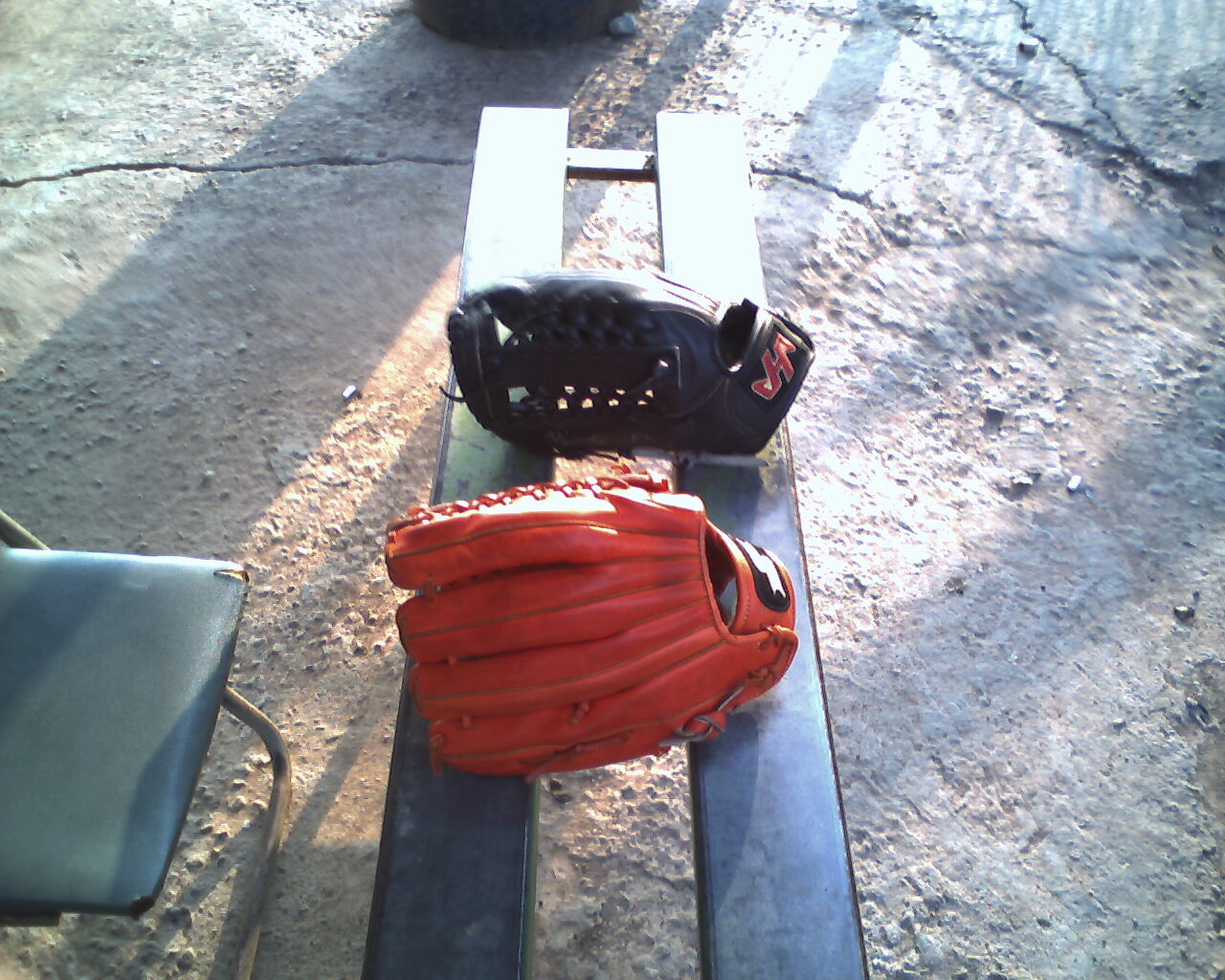The image depicts a close-up of two baseball gloves resting on a double-slat wooden bench situated on cracked concrete. The red glove, which immediately draws attention with its vibrant apple-red color and detailed stitching, is positioned at the forefront. Behind it, there is a black baseball glove adorned with red lettering; it could be mistaken for a catcher's face shield due to its placement and shape. To the left side of the image, part of a folding chair with a black seat and metal legs, possibly gold or dark gray, is visible. The scene is bathed in daylight, illuminating the bench and highlighting the rough texture of the surrounding concrete. There are no signs of greenery or people, suggesting a quiet, perhaps deserted, outdoor setting.